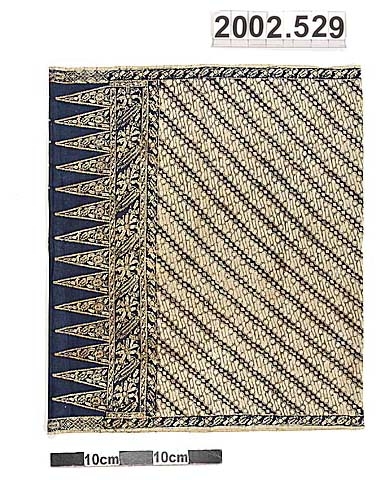The image features a centrally positioned carpet swatch with a nubby texture and a unique pattern. The swatch showcases a black, toothed pattern emerging from the left edge, transitioning into diagonal lines on a beige background. These lines create a braid-like, alternating pattern from the upper left to the lower right. The swatch has shades of black, white, yellow, tan, and varying grays. Positioned on a stark white background, the image includes the numbers "2002.529" in the upper right corner and the measurement "10 centimeters" in the white negative space between three rectangles that frame the image. Additionally, a color code is visible at the bottom left corner.